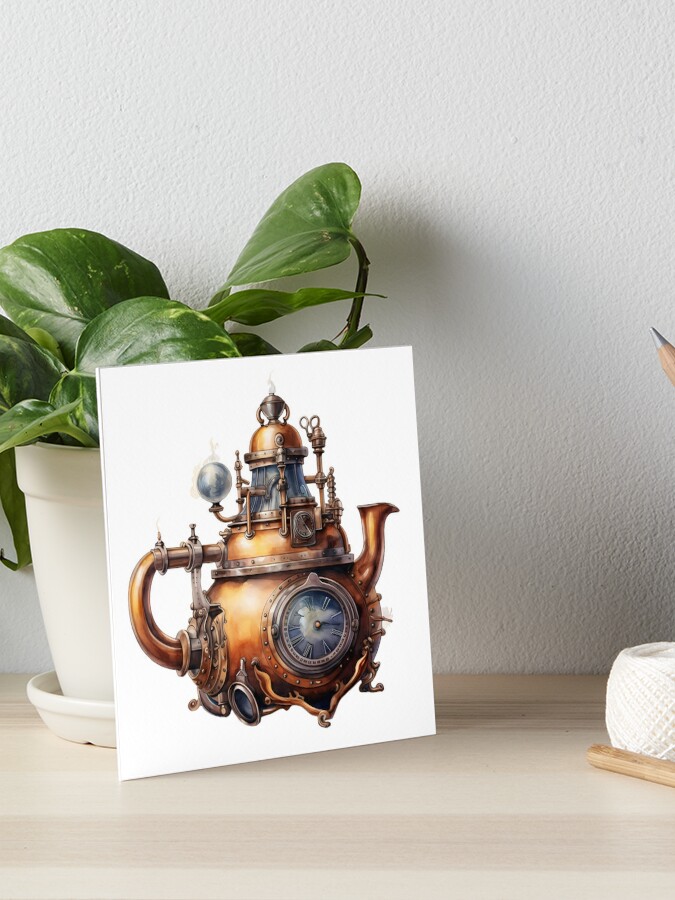The photograph depicts a small, staged scene where a modern composition focuses on a steampunk-inspired artwork. The artwork, propped against a white pot containing a lush green ivy plant, showcases a colorized image of a copper, pot-bellied teapot adorned with a clock face and various intricate mechanical elements, giving it an old-timey steam engine era aesthetic. The background features a white, painted drywall, and the items sit on a light-colored wooden surface that appears to be part of built-in furniture. Additional elements in the scene include a ball of yarn and what seems to be a large wooden pencil and the handle of another wooden object, subtly adding to the composition's detailed and ornate arrangement.